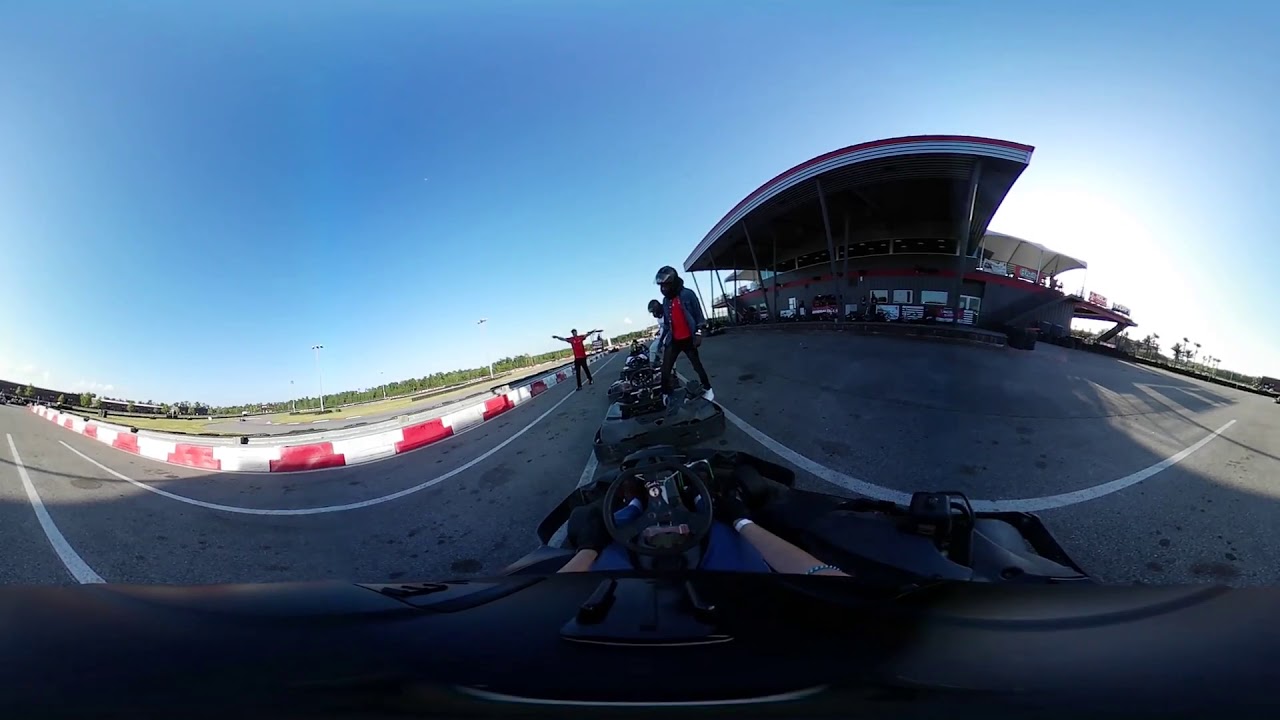The image captures a dynamic scene at a go-kart or racetrack from a first-person perspective inside a vehicle, most likely a race car or a go-kart. The driver's hands, clad in black gloves, grip a black steering wheel. In front of the vehicle, a person dressed in black pants and a red shirt stands next to another individual wearing a red shirt and denim jacket with a helmet. This second individual is standing beside a motorcycle. The asphalt road beneath them features painted markers and edge lines. To the side, a red and white roping, or perhaps a protective wall, separates the track area. There is a building with a stylistic awning, reminiscent of 1940s or 1950s architecture, possibly used for tire storage. The structure is primarily red, white, and gray. Trees are visible in the distance, adding a touch of green to the predominantly blue sky, which is clear and occupies the upper half of the image. The scene is brightly lit, indicating it is taken outdoors in the middle of the day.